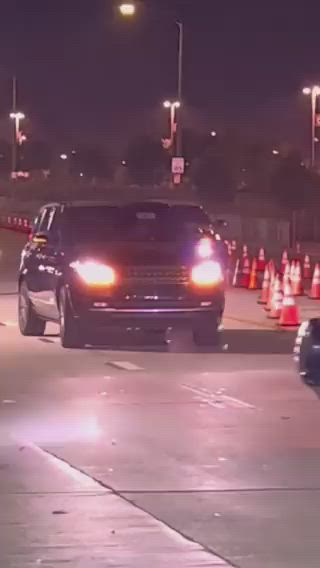The image captures a dimly lit, blurry, low-resolution nighttime scene featuring a dark blue or black small SUV with its headlights turned on. The vehicle appears to be traveling on a weathered, grayish road, possibly in a parking lot or a road under construction, indicated by the presence of numerous orange and white traffic cones lined up on the right side of the image. Another indistinct vehicle, likely a crossover SUV, follows behind. In the background, the image shows street lamps—both tall ones in the far distance and smaller ones closer to the foreground—casting light across the scene. Additionally, a barely visible speed limit sign stands on one side, its numbers unreadable in the dim light. An ambiguous blackish object, possibly another car or obstruction, appears in the foreground to the right, adding to the overall complex and nighttime atmosphere of the scene.